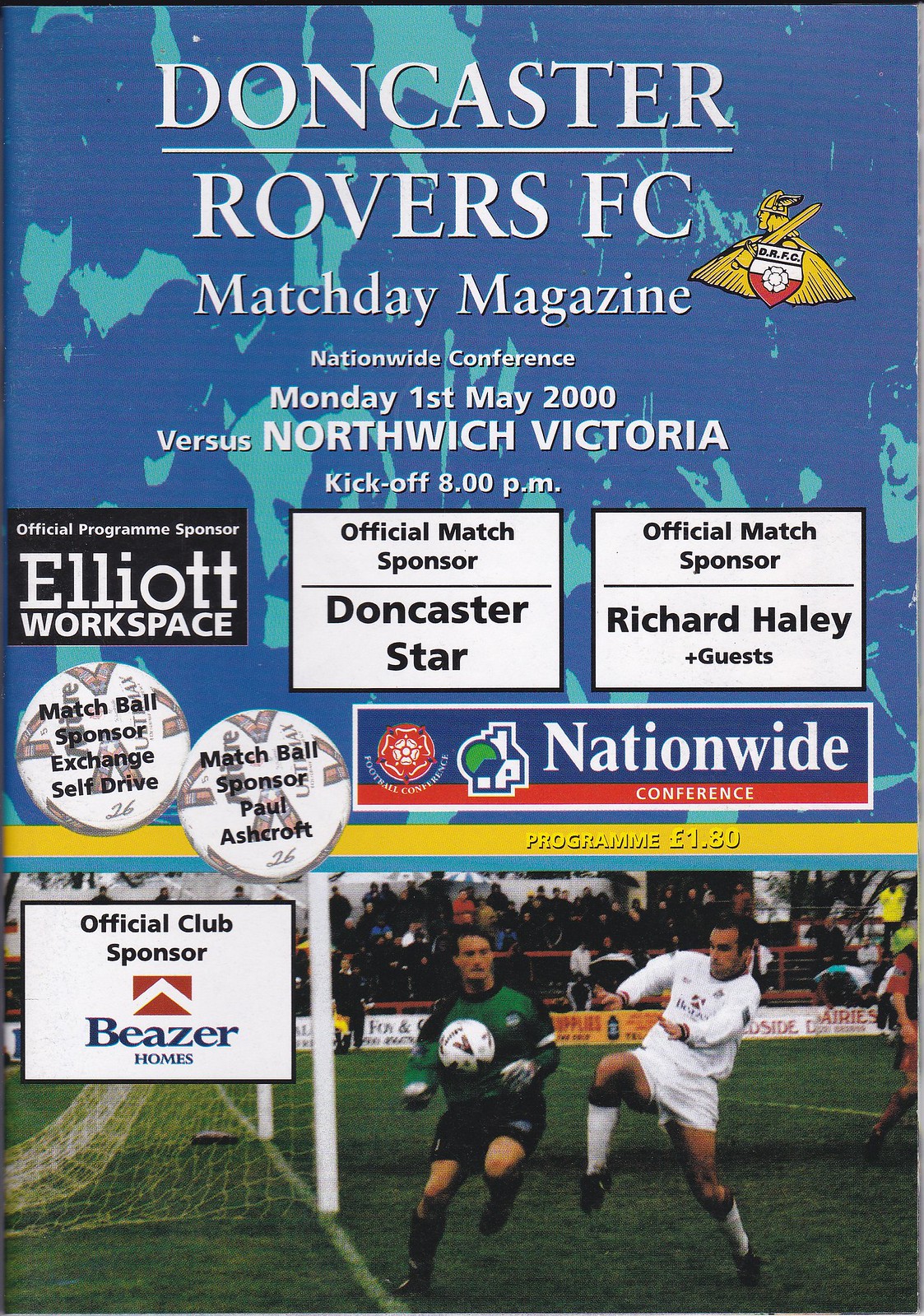This is a detailed poster promoting a soccer event, mainly emphasizing a Match Day magazine for a game between Doncaster Rovers FC and Northwich Victoria in the Nationwide Conference. The match is scheduled for Monday, 1st May 2000, with kickoff at 8 PM. The top of the poster prominently features the title "Doncaster Rovers FC Match Day Magazine," along with the game details. The background of the poster has a green and blue theme. Notably, there's a depiction of a yellow Viking with a cape, wielding a sword over its left shoulder, representing the Doncaster Rovers Football Club.

Below the match details, there are three white sponsor boxes: the first one on the right highlights "Official Program Sponsor: ADR Workspace," the second in the middle mentions "Official Match Sponsor: Doncaster Star," and the third on the left indicates "Official Match Sponsor: Richard Harley and Guests." Furthermore, a sign mentioning "Nationwide Conference" is included below the sponsors’ section.

At the bottom of the poster, an image showcases two soccer players battling for the ball near the goalpost. The player on the left is wearing a green jersey, while the player on the right sports a white jersey, both actively engaged in the game. The program is priced at one pound and eighty pence. The use of blue color and thematic elements like badges and additional sponsor details complement the overall aesthetic of the poster.